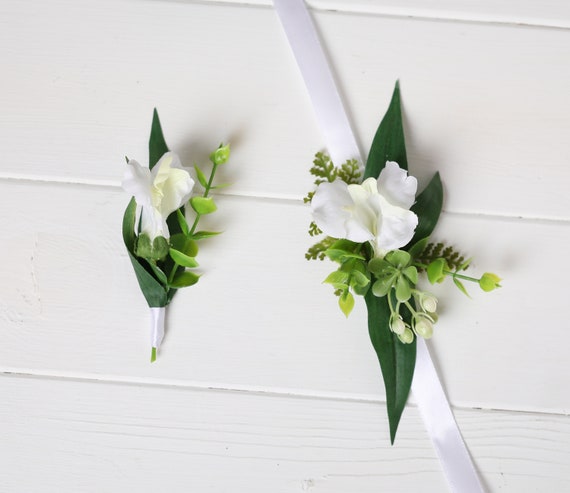In this indoor, full-color photograph, two delicately arranged corsages are pinned against a white, lacy-surfaced background, set on horizontal, right-tilting wooden or painted plastic slats. The image, which is square with no border, features a striking juxtaposition of floral beauty. The corsage on the left is slightly smaller, showcasing a single white flower cradled by a dark green leaf, with sprigs of smaller green leaves and a tiny white ribbon securing the base. The larger corsage on the right is more elaborate, adorned with additional green leaves, more sprigs, and a distinctive white ribbon elegantly woven from top to bottom. Both corsages, with their intricate arrangements and the underlying wooden board's textured surface, create a harmonious and artistic display.